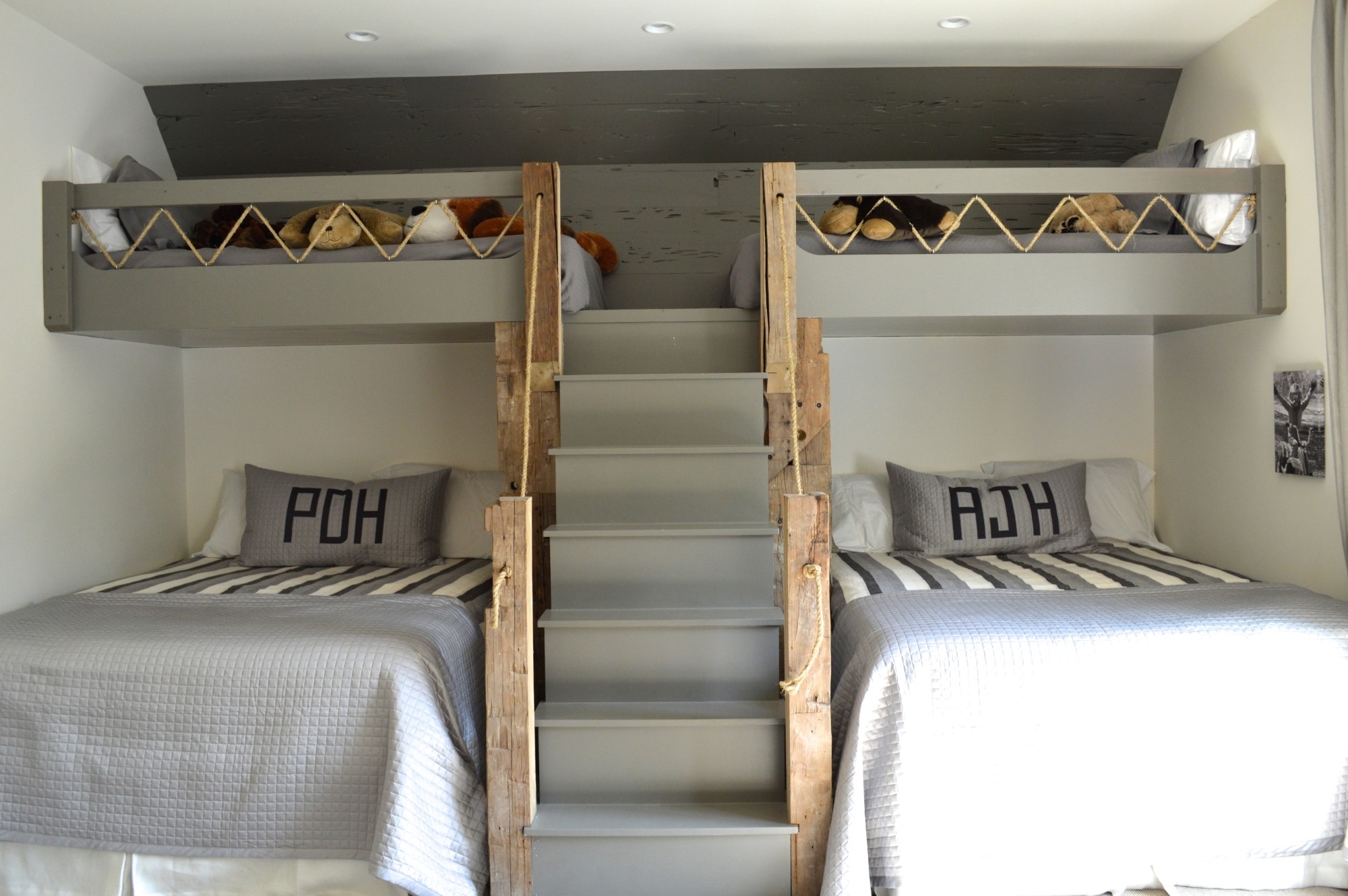This color photograph showcases a cozy, well-organized tiny house bedroom featuring a unique bunk bed setup. Centered in the room, a staircase with gray steps and wooden posts leads up to a loft area, flanked by twin beds below. The staircase, comprising seven steps, is decorated with a rope banister on each side for a nautical touch. 

On the ground level, the twin bed to the left is adorned with a gray pillow monogrammed 'PDH' and gray and white striped sheets and blankets. Similarly, the twin bed on the right features a gray pillow with the initials 'AJH' and matching bedding. Both beds are positioned against white pillows for added comfort.

Above, in the loft, two smaller twin beds rest on either side of the staircase, featuring railings with rope spindles for safety. These loft beds are decorated with stuffed animals, adding a playful and homey feel to the room. The walls are painted a soothing light gray, complementing the overall color scheme and adding to the room's charm.